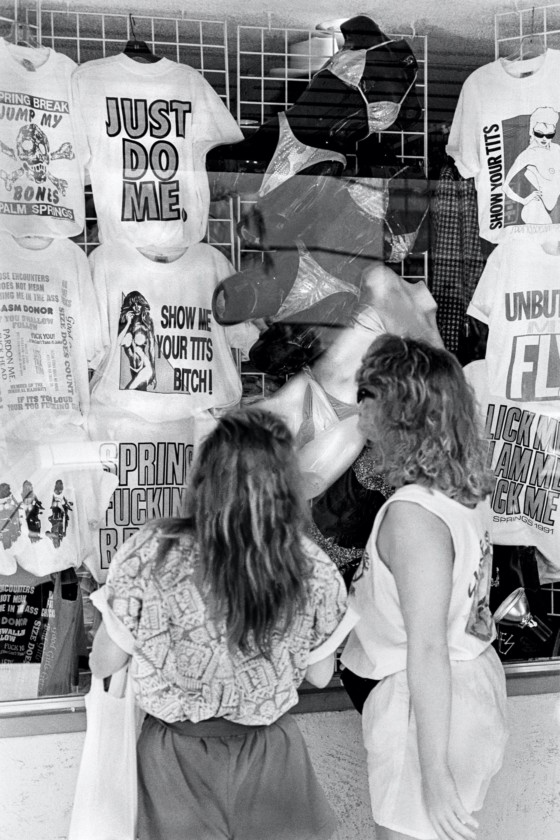In this black and white photograph, two women stand with their backs to the camera, looking at a display of adult-themed t-shirts and bikinis. One of the women, who is wearing sunglasses, a tank top, and shorts, stands slightly sideways, allowing a partial view of her face. The other woman is dressed in a short-sleeve shirt. They are positioned behind a counter that showcases various t-shirts, some of which bear provocative slogans such as "Just Do Me" and "Show Me Your Tits Bitch." The t-shirts are predominantly white and hang above and around several bikinis. The window display has a vintage feel, reminiscent of 1980s fashion. The mannequins displaying the bikinis vary in color, with some being black and others lighter. The women appear to be absorbed in deciding which items to purchase in this intriguing and risqué storefront.